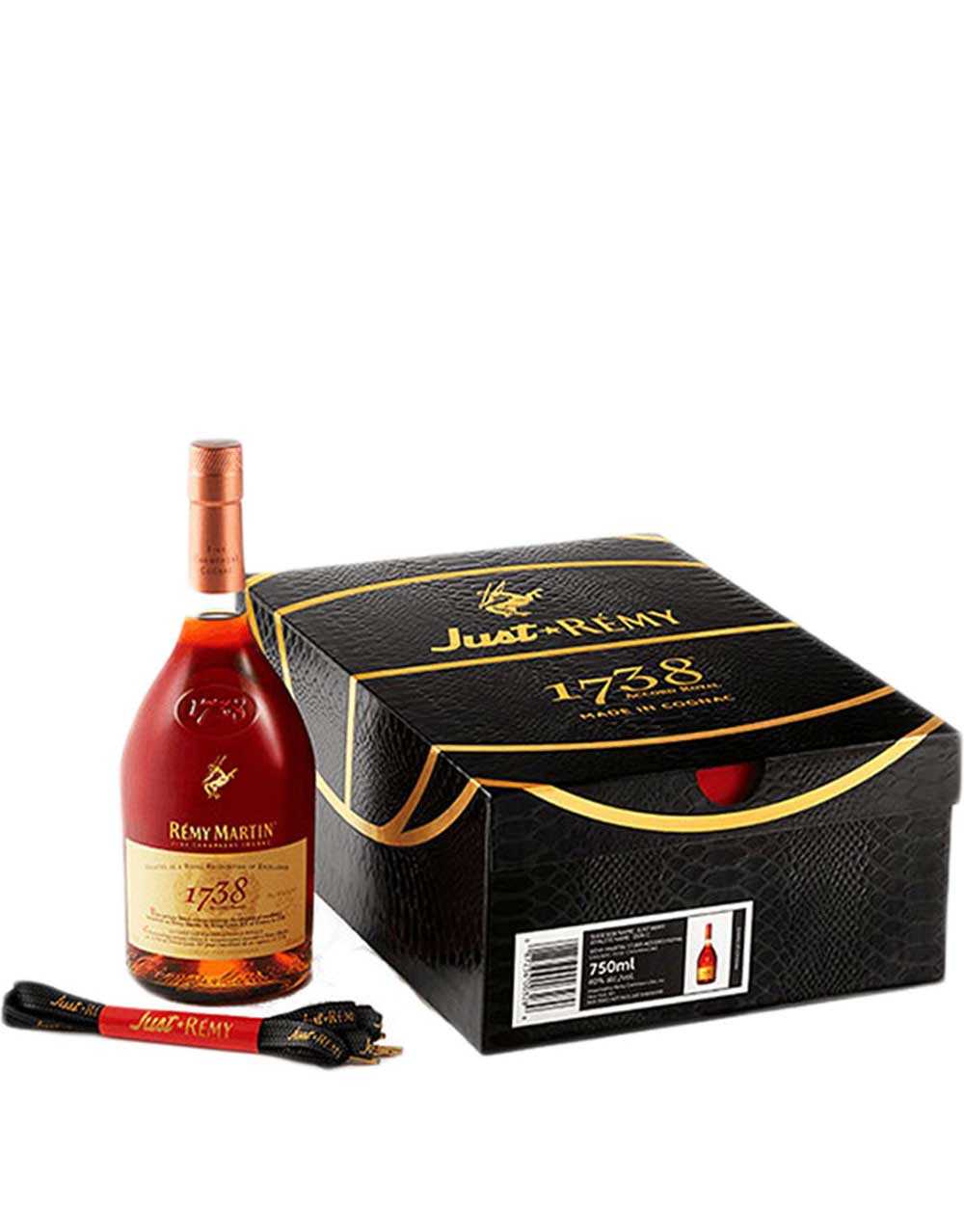This image showcases a luxurious promotional setup on a pure white background, featuring an upscale bottle of liquor and an ornate box. The rectangular box, designed to resemble a shoebox, is black with an elegant gold leopard-snake print pattern and multiple textures that mimic leather. It prominently displays the brand name "Just Remy" in gold lettering across the top, along with "1738" and "Made in Cognac." The front side of the box includes a gold band, an outline of a basketball, and a barcode, with "750 milliliters" printed in white text beside a picture of the bottle.

To the left of the box, a bottle of Remy Martin stands regally. The bottle is a deep reddish-orange hue with a gold top and a series of gold labels. The top label reads "Remy Martin," while the central gold label repeats "1738." Below the bottle, there appears to be a folded black ribbon with gold lettering stating "Just Remy," held together by a red label. Adjacent to it lies what looks like a package of black shoestrings with gold tips, adding to the sophisticated aesthetic of the display. The overall presentation exudes an air of exclusivity and high-end craftsmanship.